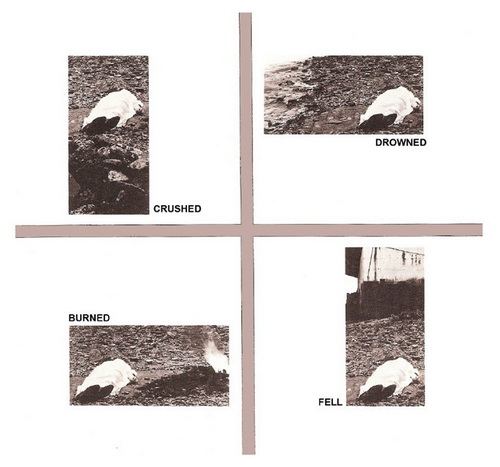The image is divided into four quadrants, separated by a beige plus sign in the center. Each quadrant has a black-and-white photograph depicting a similar creature lying on the ground. The images are slightly different and each has a unique caption in black text. In the upper left, the creature is next to a few rocks and the caption reads "crushed." The upper right shows the same creature near water, labeled "drowned." In the bottom left, the creature appears next to flames, with the caption "burned." The bottom right image shows the creature lying in front of a building, labeled "fell." Each photograph represents a different way the creature might have met its demise, with the overall aesthetic suggesting old, somber scenes.